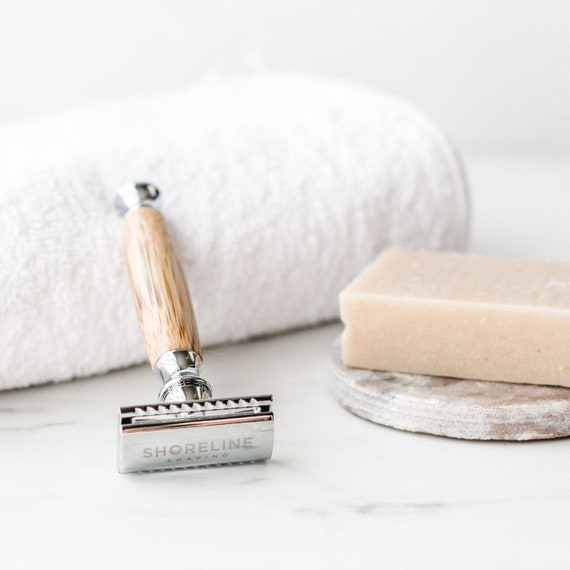In this elegantly styled image, a collection of high-end shaving accessories is artfully arranged on a sophisticated white and gray veined marble surface. To the left, a plush, premium-quality white towel is neatly folded, providing a luxurious backdrop. Resting against the towel is a high-class, old-fashioned razor featuring a wooden handle and a gleaming silver head, inscribed with "Shoreline Shaving." The razor, exuding elegance and refinement, has a blade already inserted into its head. On the right, a thick, off-white bar of soap lies pristinely on a round soap dish or coaster, which appears to be crafted from a gray and white material possibly marble. The overall presentation suggests a high-end advertisement, likely for a luxury hotel or premium shaving products, characterized by an understated yet sophisticated color palette and meticulous attention to detail.